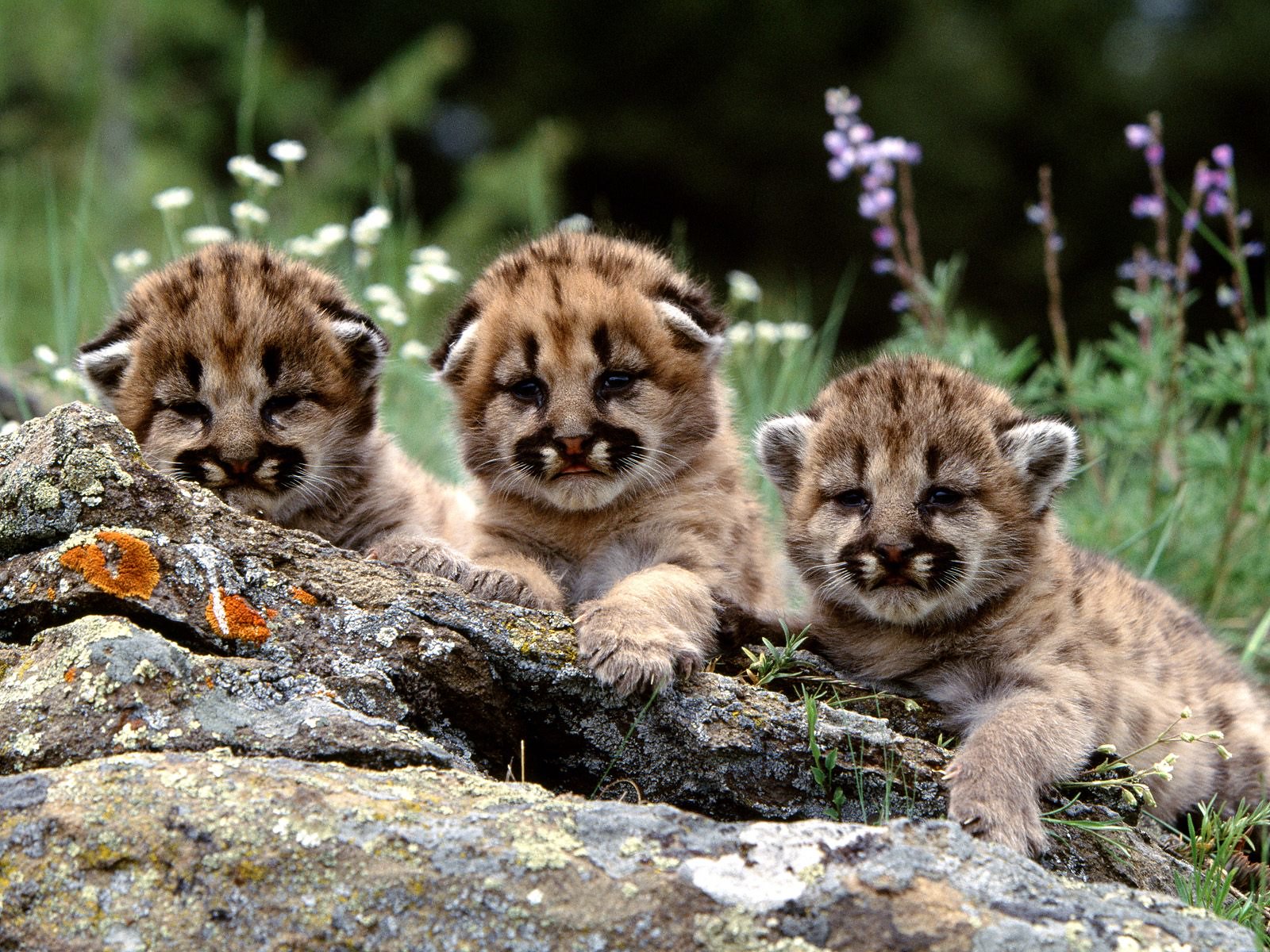This captivating photograph features three young wildcat cubs, possibly jaguars or cheetahs, with distinctive spots that aid in their camouflage. The cubs, appearing siblings, are nestled against a prominent, light gray rock formation adorned with an array of colorful lichen, including notable orange patches. Their expressive faces are directed towards the camera, showcasing their innocent gaze with eyes wide open. The two cubs on the left have their ears flattened, while the one on the right has its ears perked up, enhancing their endearing appearance. In the blurry background, delicate white and light purple wildflowers can be seen, adding a splash of color to the verdant green surroundings. The entire scene is framed by a shadowy area hinting at dense foliage or trees beyond, enriching the natural ambiance of their habitat.